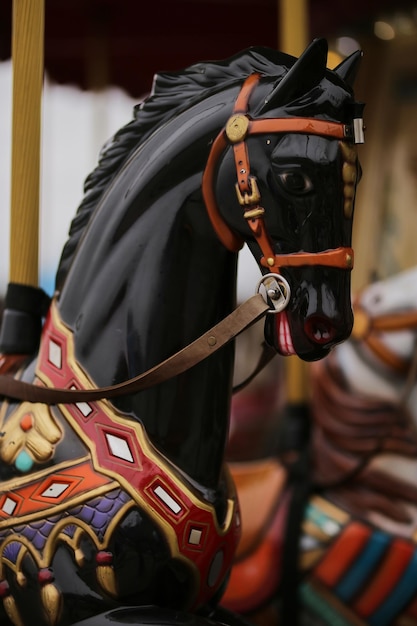This close-up photograph captures a black ceramic toy horse that is part of a carousel ride, likely found at a carnival or fair. The image shows a detailed side view of the horse, revealing its head and part of its body. The horse, which appears to be slightly smiling with visible light pink teeth, is adorned with a vibrant red halter featuring gold straps. A yellow spiral pole is attached to the horse, extending upwards as part of the carousel structure. Other elements of the carousel are visible but blurred in the background, including what seems to be a white horse. The black horse displays intricate designs in red, orange, blue, and purple—likely representing a decorative saddle or blanket. The reins, made of brown leather, trail back from its head, providing handles for riders. The precise craftsmanship of the ceramic material gives the horse a polished brown sheen, enhancing the overall nostalgic charm of this fairground attraction.